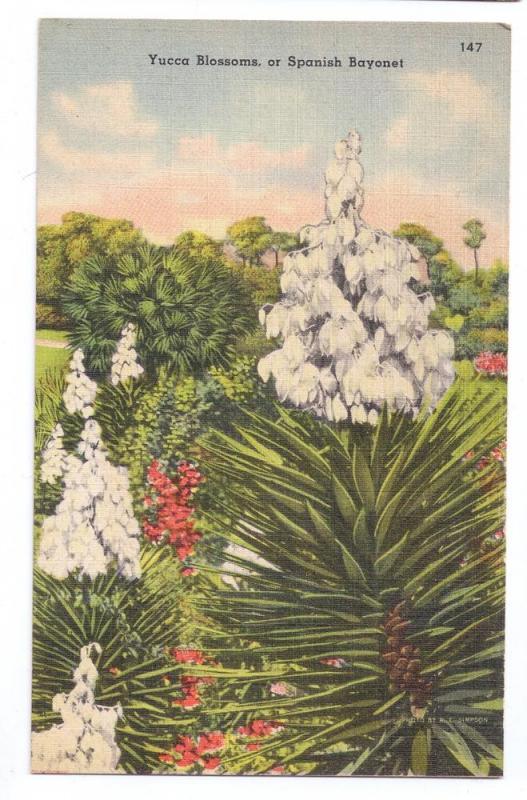This full-color, vertically rectangular postcard features an artistic depiction, possibly created with ink or paint, titled "Yucca Blossoms or Spanish Bayonet" at the top. In the upper right-hand corner, the number 147 is visible. The postcard showcases an outdoor scene dominated by a yucca plant, characterized by its dark green, spiny leaves and white, drooping flowers grouped in triangular clusters. Interspersed among the yucca blossoms are vibrant red flowers. The background includes green trees, additional shrubs, and a sky that transitions from blue to hints of white and pink clouds. To the upper right, a tall tree stretches into the sky, contributing to the natural scenery. The composition suggests a balance of detailed plant life against a tranquil sky, capturing the essence of this yucca landscape.